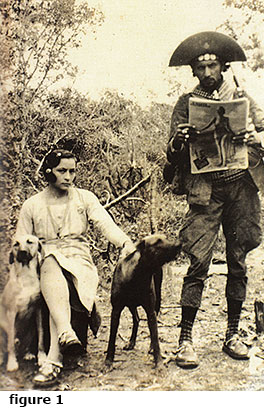This sepia-toned photograph, reminiscent of the 1930s or 1940s, captures a detailed scene. A woman, with her hair styled in pin curls and adorned with two hair bobs, is seated in the center. She wears a white suit with a tie around the waist and sturdy shoes that are neither clogs nor sneakers. The woman directs a slight side-eye and upward glance, with one hand resting on each of the two dogs flanking her — likely Rhodesian Ridgebacks or mixed breeds, one lighter-colored to her left and a darker one to her right. To the far right stands a man who is intriguingly dressed in what appears to be either a pirate costume or golf attire. He sports a semicircle-shaped hat and is holding up a magazine, ostensibly featuring an image of a naked or scantily clad person. The background is filled with trees or bushes, adding to the vintage outdoor setting. Below the image is a caption that reads "Figure 1," suggesting this photograph might be an excerpt from a book or an old document, further adding to its historical charm and ambiguity.